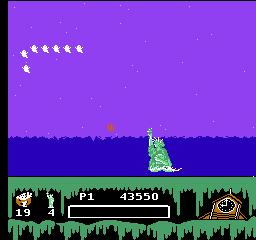This image depicts a scene from an older, pixelated video game with a distinctly retro aesthetic. The background is predominantly purple, indicating a twilight sky dotted with seven stars—five aligned horizontally and two descending from the left. A notable feature in the image is the top of the Statue of Liberty emerging from what appears to be dark blue water, located slightly off-center to the right. Near the statue, a small red object is visible in the sky, adding a splash of color to the scene.

The lower portion of the image is divided into a green section layered above a black, possibly subterranean, area with dripping green highlights. On the left side of the screen, the number 19 in white is displayed above a small Ghostbuster icon, with the number 4 accompanied by a miniature Statue of Liberty below it. Centrally, the text "P1 43550" is prominently featured in white, with a black rectangle beneath it. To the right, there is a small image resembling a wooden clock. The overall image exudes the charm of retro video games, reminiscent of titles like "Oregon Trail."